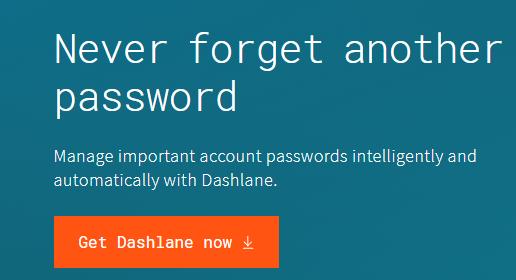This image features a section of a website dedicated to promoting Dashlane, a password management tool. The primary focus is a large, cyan-colored rectangular box, with the background hue being a blend of blue and green in a dark cyan shade. 

At the top of the box, in bold white text, is the title "Never forget another password," with "Never" capitalized and the rest in lowercase, devoid of any punctuation. Beneath this headline, a smaller, white text reads: "Manage important account passwords intelligently and automatically with Dashlane," ending with a standard period.

Situated below this informative text is a prominent, bright orange button that closely borders on neon but is slightly darker. The button displays the CTA (Call to Action) text "Get Dashlane now" in all capital letters, accompanied by a download icon. 

The entire textual content is white, standing out vividly against the contrasting cyan background. The screenshot appears slightly off-center, with more visible space on the left side compared to the right, indicating an imperfect cropping job.

This image effectively highlights key features of Dashlane while presenting a clear and visually appealing call to action.